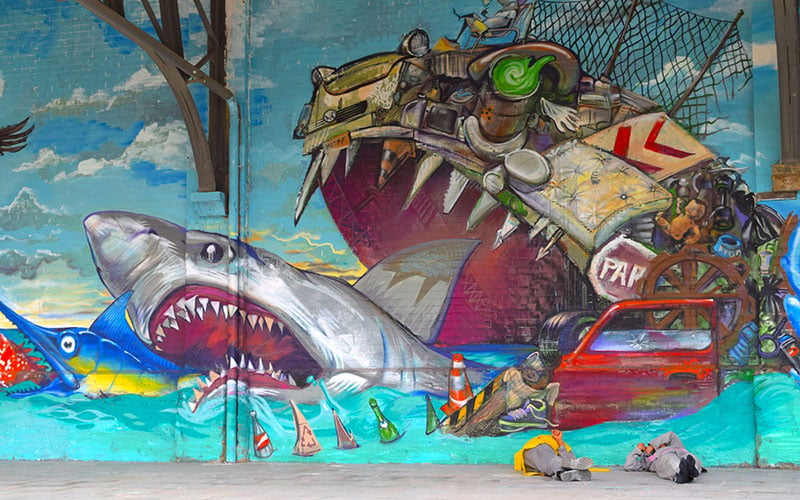The image captures a vividly colored mural on an outdoor wall, possibly under a bridge with visible arched support beams. The mural presents a striking ocean scene rendered in a cartoonish style. Central to the mural is a dramatic depiction of the ocean's food chain disrupted by pollution: A large great white shark with menacing teeth is consuming a marlin or swordfish, which in turn, is swallowing a smaller redfish. Overshadowing this scene, a monstrous figure composed of ocean trash, like car doors and bottles, is devouring the shark, suggesting the destructive impact of pollution. The waters in the mural are a bright teal blue, adding vibrancy to the artwork. In the foreground, two individuals wearing gray clothing, one with a yellow top, are laying on a silver sidewalk or street, their heads against the mural. The overall theme underscores the devastating effect of pollution on marine life, illustrating that trash ultimately defeats all fish.